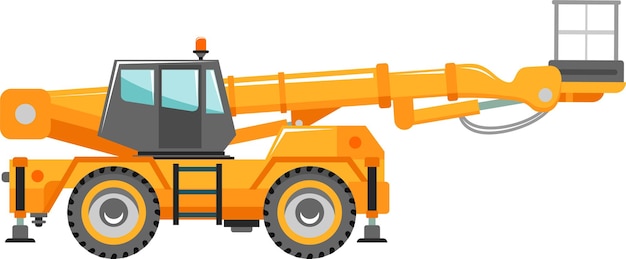This is a detailed, cartoonish drawing of a yellow-orange, wheeled work lift platform. The image primarily showcases an elevated hydraulic lift with a multi-level telescoping arm, designed for reaching high places. The base of the platform is equipped with leveling hydraulics at each corner to ensure stability. The tractor-like base is orange with large gray tires, accented by orange centers, which match the primary color of the machinery. A flashing amber light is positioned atop the cab, which is a gray compartment hosting the controls such as buttons, levers, and a steering wheel. The lift arm extends upwards, leading to a gray and black standing platform or cage where workers can safely stand. The overall aesthetic is cartoon-like, with simplified, bold color uses: the machinery is predominantly yellowy-orange while the cab, platform, and tires are gray, with the background left white for emphasis. The image meticulously details the equipment's structure and functionality, highlighting safety features like the stabilizing prongs and the design of the lift’s arm and carriage.